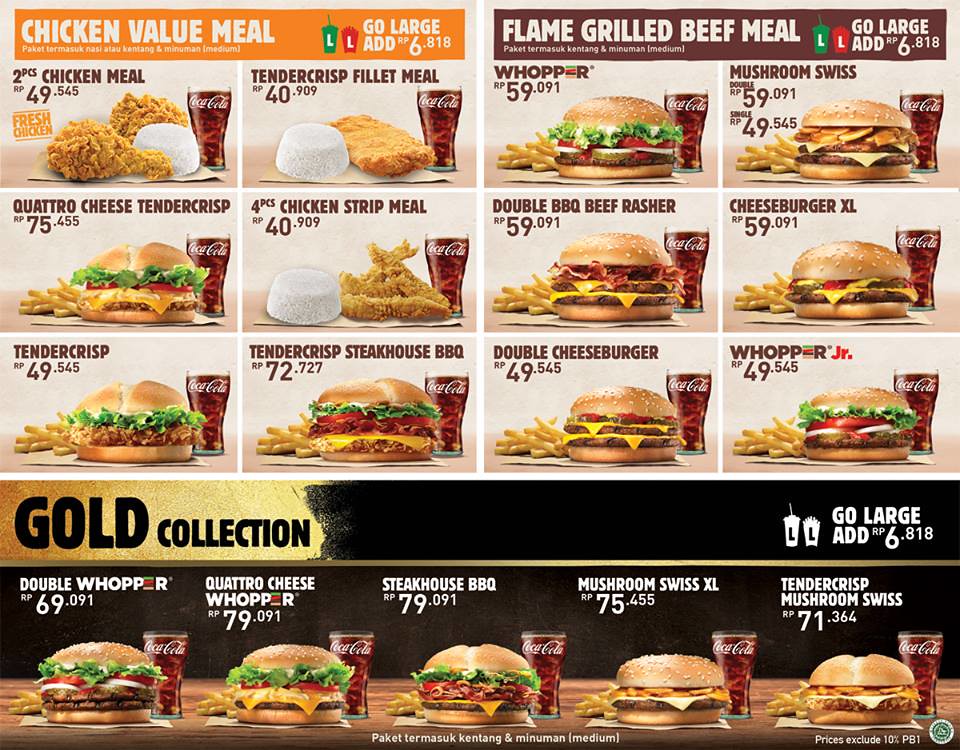This image is an advertisement for an Indian Burger King menu, featuring a detailed and vibrant layout showcasing various meal options. At the top left, the section is labeled "Chicken Value Meal" and displays six different chicken dishes, including options like Tender Crisp, Filet Meal, Quattro Cheese, and Chicken Strip Meal. Accompanied with high-quality images of meals featuring chicken pieces, sides like rice or biscuits, and a glass of Coca-Cola, the prices are listed in Rupees (RP). 

On the right side of the menu, another section highlighted is the "Flame Grilled Beef Meal," offering six variations including the Whopper, Mushroom Swiss, Double BBQ Beef Fresh, and Cheeseburger XL. The menu indicates the option to upgrade to a large meal for an additional cost.

At the bottom of the menu, set against a dark background with gold highlights, the "Gold Collection" features premium selections such as the Double Whopper, Quattro Cheese Whopper, Steakhouse BBQ, and Mushroom Swiss XL. 

The colors used throughout the menu include gray, orange, green, red, brown, tan, white, and yellow, creating a vibrant and appetizing visual appeal. The overall layout is well-spaced, detailed, and clearly intended to entice and inform customers with the high-quality images and detailed meal descriptions.